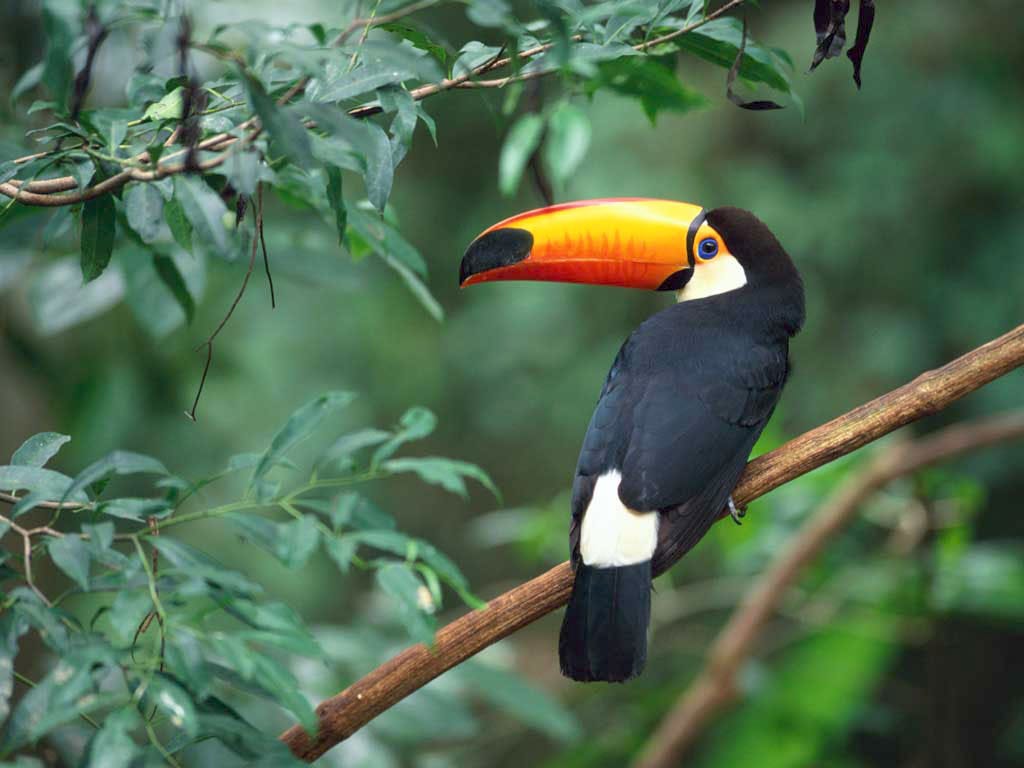The image showcases a close-up view of a toucan perched on a brown limb, set against a muted green background with out-of-focus leaves. The toucan, occupying the middle to the right side of the picture, commands attention with its striking appearance. Its head is adorned with a bold black hue, transitioning to a patch of white on its face where intense blue eyes, outlined in orange-yellow, peer back at us. The bird's prominent yellow-orange beak, thick and curving, features distinctive black markings at the tip and base. Below its face, the toucan's body is primarily black, contrasting sharply with white patches near its tail feathers. The composition emphasizes the toucan's vivid details and vibrant colors, making it stand out amidst the natural, leafy branches around it.